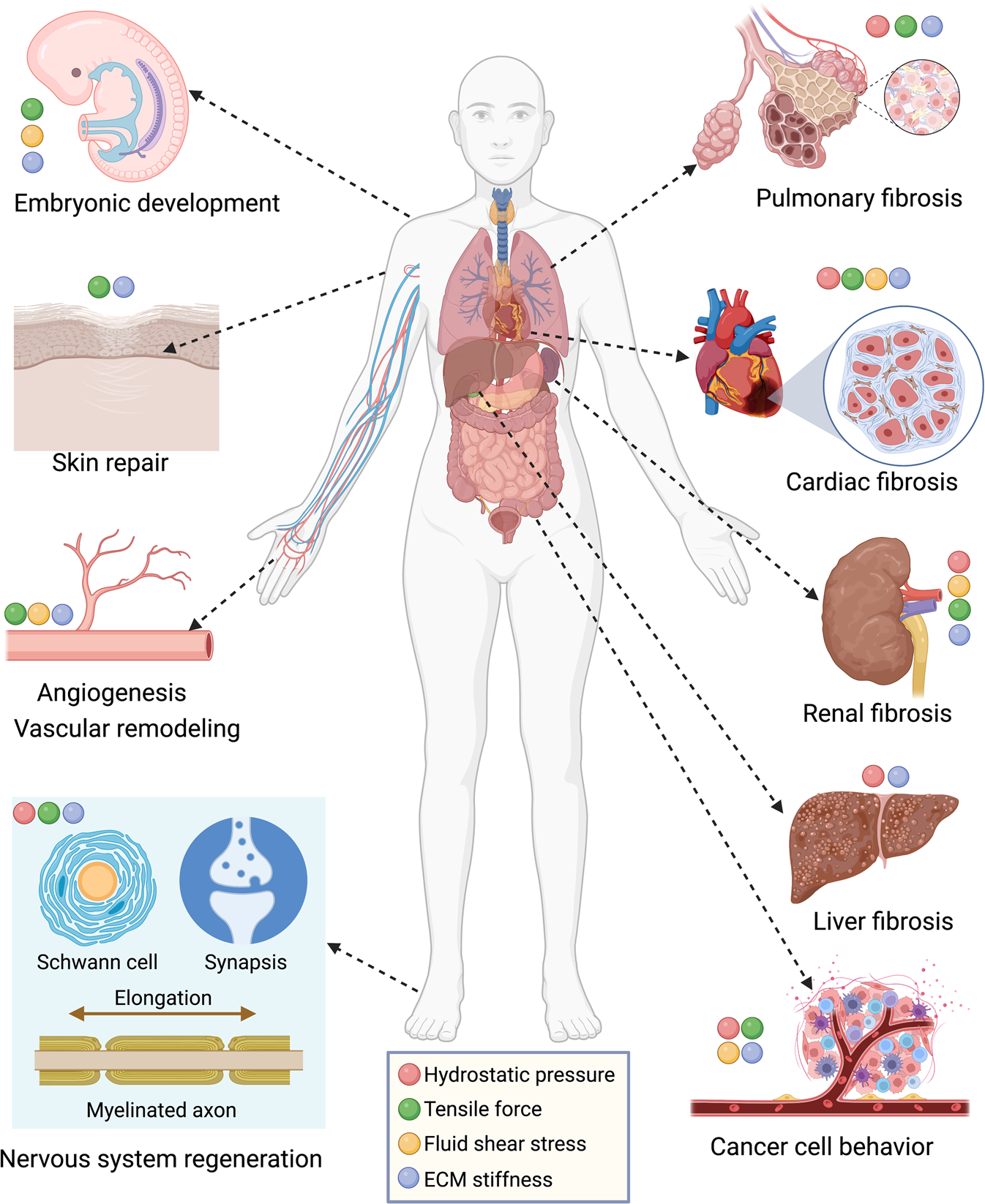A detailed scientific and educational illustration prominently features a gender-neutral, faceless human body outline against a white background, revealing internal organs from the throat to the bladder. The organs inside the torso are color-coded and thoroughly detailed. Dotted lines connect these organs to larger, close-up depictions with annotations describing specific medical conditions. Notably, the lungs are linked to pulmonary fibrosis, the heart to cardiac fibrosis, the kidneys to renal fibrosis, and the liver to liver fibrosis. On both sides of the body, rich details unfold.

On the left side, annotations highlight various biological processes: embryonic development connected to the shoulder, skin repair from the other shoulder, and angiogenesis and vascular remodeling from the hand's blood vessels, which are distinctly blue and red to depict veins and arteries. Further down, another section addresses nervous system regeneration, including myelinated axons elongation, Schwann cells, and synapses.

On the right side, at the bottom, a section labeled "Cancer Cell Behavior" delves into cellular mechanisms. 

Supplementing this, at the bottom center, a blue square encloses key biomechanical properties illustrated with different colored bullet points: red for hydrostatic pressure, green for tensile force, yellow for fluid shear stress, and blue for ECM stiffness.

This comprehensive depiction integrates anatomical visuals with pathological and physiological annotations, creating an intricate and informative resource.